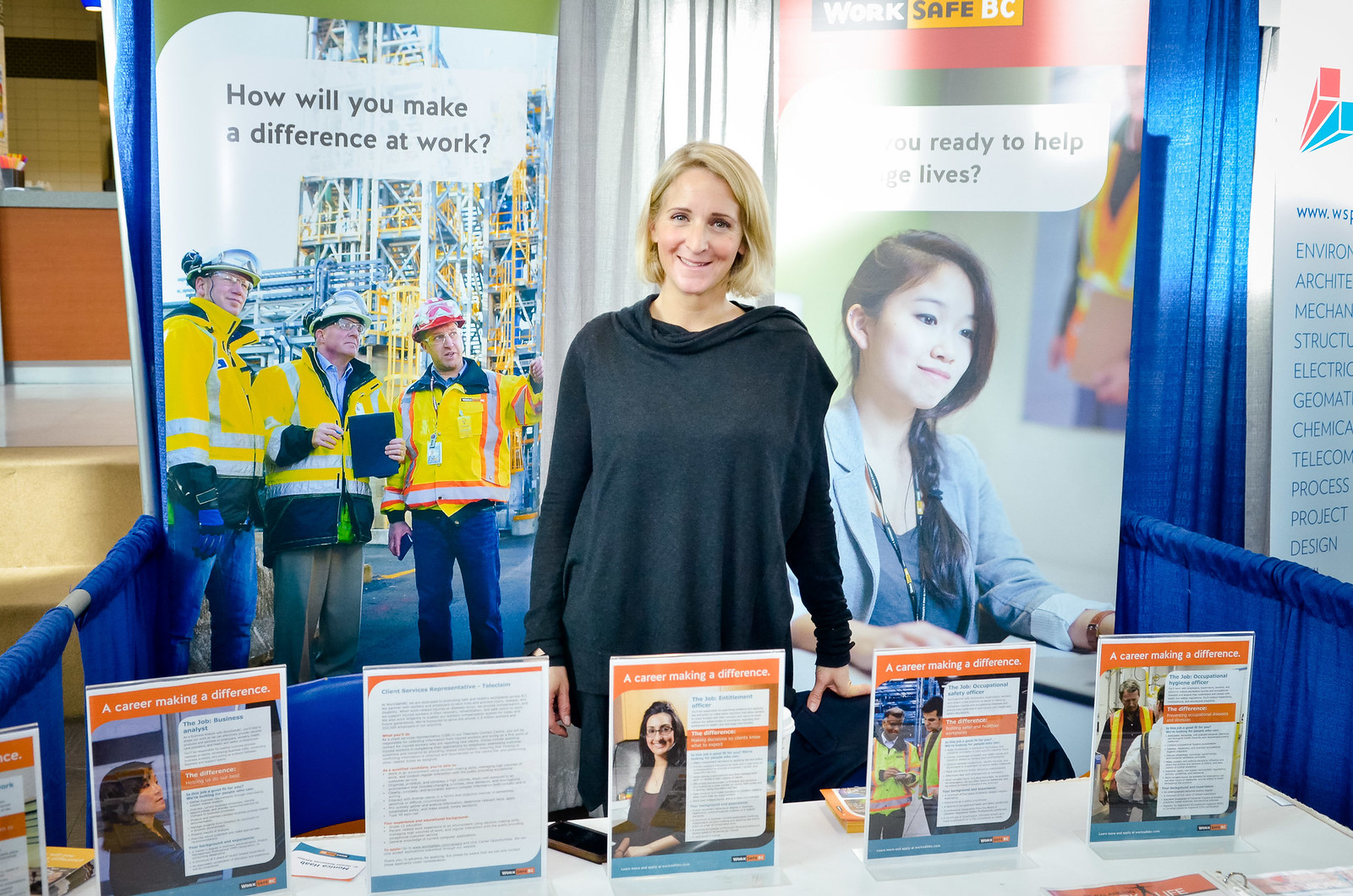The image captures a woman, approximately 25 to 30 years old, standing behind a table at a convention or expo. She is a smiling white woman with short blonde hair, wearing a black sweater. Her table is laden with informational brochures about careers in workplace safety and making a difference. Behind her are multiple banners: one features a construction crew in helmets and reflective vests on an oil rig, accompanied by the text "How will you make a difference at work?"; another banner displays an Asian girl working on a laptop, labeled "WorkSafe BC." A third banner shows a girl with braids and a message potentially about readiness to help and save lives. These elements suggest the event is focused on work safety and networking, potentially highlighting various occupational safety careers, possibly relating to OSHA standards.